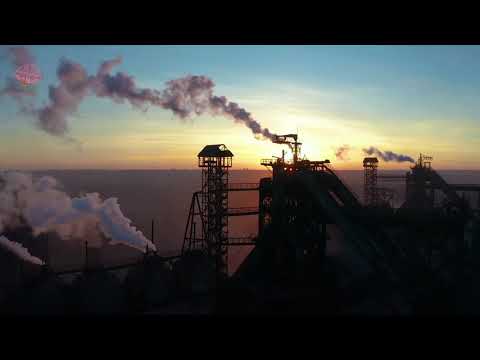The photograph captures an industrial complex set against the backdrop of either a sunrise or sunset, with the sun positioned at the horizon, casting an orange hue on the water and the sky, which transitions to light blue with some cloud cover. The image is in a horizontal rectangle format with black letterboxing bars at the top and bottom. The foreground features a series of dark, shadowed metal scaffolding, towers, and possibly silos, interconnected by bridges and some angled elevators or escalators. There are at least three to four smokestacks emitting pillars of smoke. Among the towers, one particular area has a reddish tint, possibly illuminated by the sun’s light. The industrial complex appears to be located at the edge of a large body of water, likely an ocean, contributing to the dramatic, serene yet industrious atmosphere of the scene. No people are visible in this stark, mechanical landscape, enhancing the focus on the monumental structures silhouetted against the twilight sky.